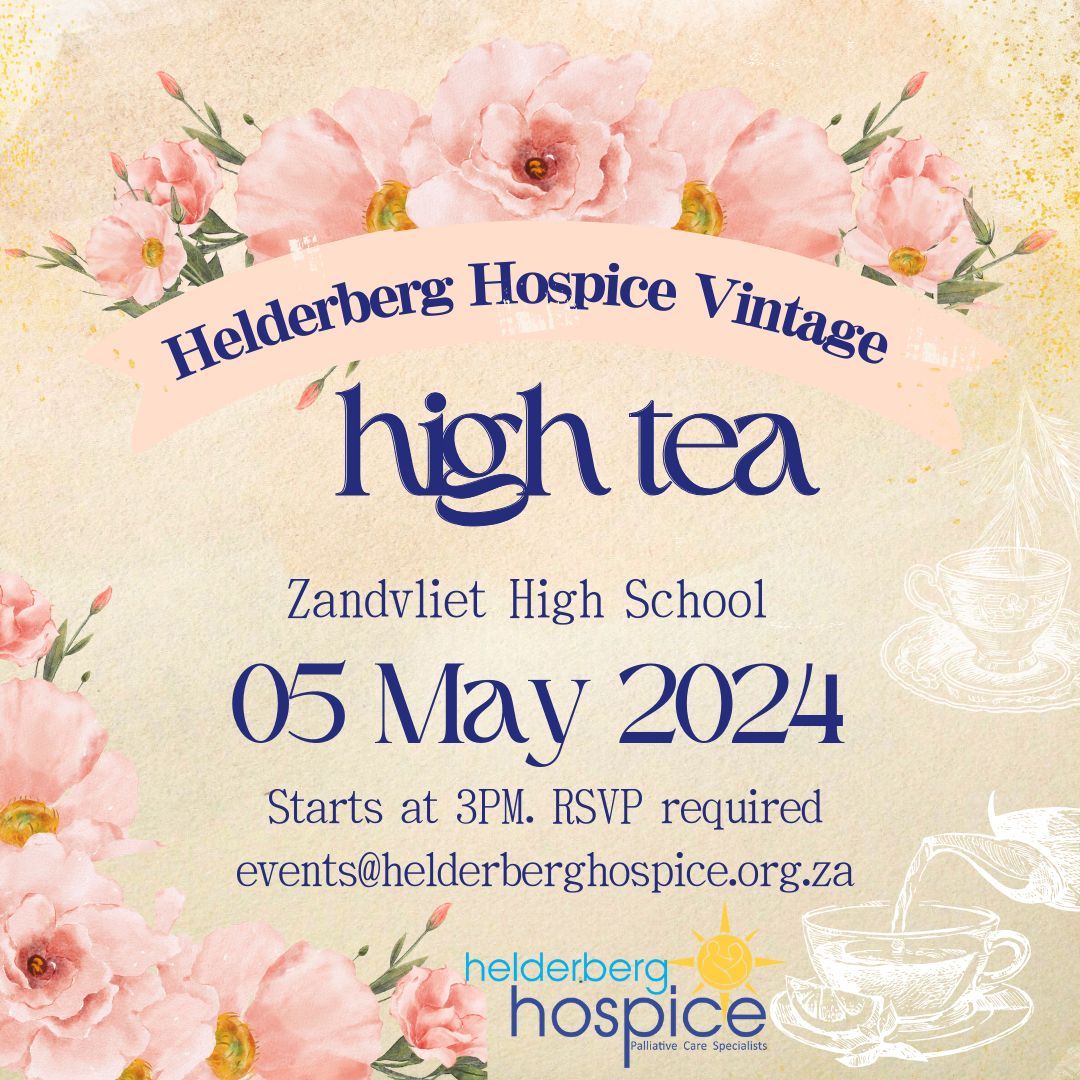The poster features a light tan, almost beige, background adorned with elegant drawings of tea cups and a tea pot, sketched in white ink. At the top, there are delicate pink flowers. The poster's heading announces "Hildebrandt Hospice Vintage High-Tea" followed by details of the event: "St. Vignette High School, 5th May 2024, starts at 3pm. RSVP required." It also mentions the event's website as "hildebrandthospice.ca." At the bottom, there are more pink flowers on the left, similar to those at the top, and on the bottom right, an illustration of a kettle pouring drinks into a cup. The poster emphasizes the event hosted by Hildebrandt Hospice, known for their palliative care services.